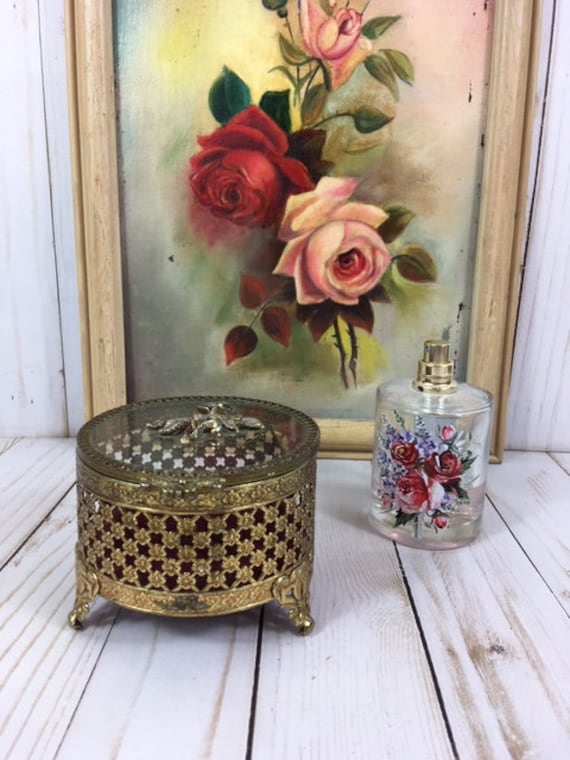The photograph depicts a rustic setting featuring a couple of products displayed on what appears to be a wooden surface with a white wood, brown-grain design. The backdrop consists of matching white wooden planks, which complement the rustic ambiance. Central to the image is a framed painting on the wall, displaying a floral motif with roses of various colors—pink on the bottom right, red on the left, and another pink rose on the top—set against a light brown, greenish-yellow background.

Foregrounding the painting, on the wooden surface, sits a clear glass perfume bottle adorned with rose patterns and a silver spray top. To the left of the bottle, there's an ornate circular gold container designed to hold jewelry, complete with intricate tripod legs and decorative notches along its sides. The composition of the photograph exudes a vintage charm through the harmonious blend of rustic textures and elegant details.